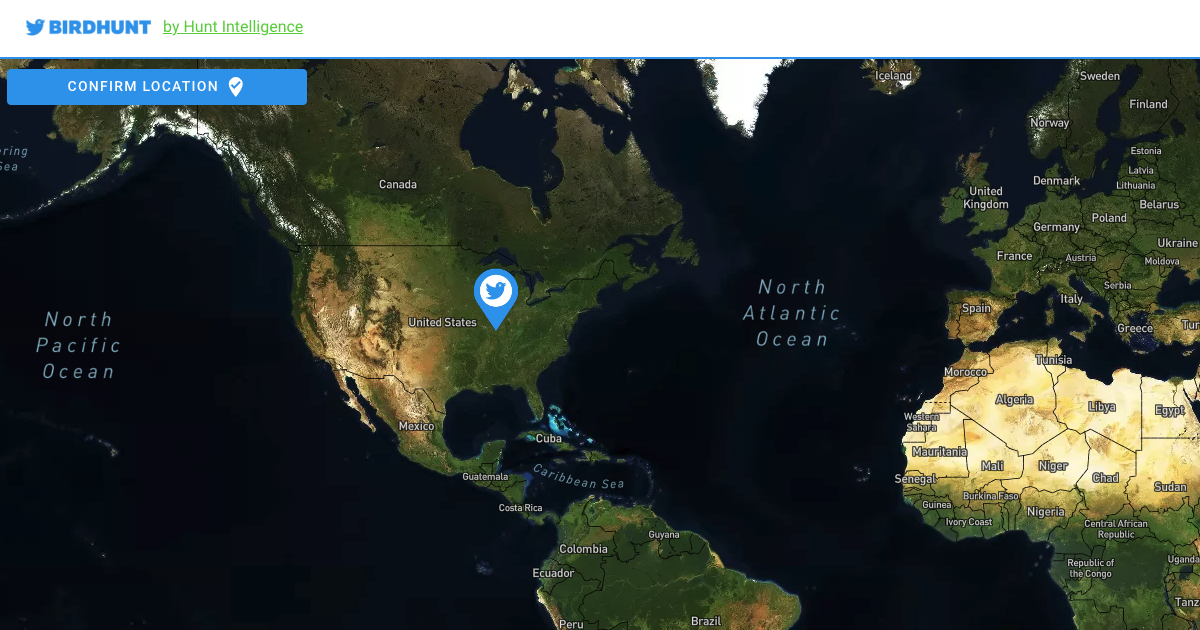This is a detailed screenshot of an application interface titled "BIRD HUNT" displayed prominently at the top in all capital letters with a blue color scheme. To the left of the title, there is a blue bird icon flying to the right, symbolizing the "Bird Hunt" theme. The application is developed by "Hunt Intelligence."

The main section of the screenshot features a large, partially-displayed world map with the text "Confirm Location" overlaid. On this map, several geographic areas and countries are labeled. The focus of the map includes regions such as the North Pacific Ocean, Canada, the United States, and parts of Mexico and Central and South America, including Cuba, Guatemala, Costa Rica, Colombia, Ecuador, Peru, Brazil, and the North Atlantic Ocean.

A prominent location pin marked with the blue bird icon from the logo is placed in the southern United States, indicating a point of interest.

At the top of the map, various European countries are visible, including Iceland, Sweden, Finland, Norway, Estonia, Latvia, Lithuania, Denmark, United Kingdom, Germany, Poland, Belarus, France, Austria, Ukraine, Moldova, Serbia, Italy, Greece, and Spain. Adjacent to Europe, North African countries such as Morocco, Tunisia, Western Sahara, Algeria, Libya, and Egypt are also labeled.

Furthermore, several countries in West and Central Africa are listed, including Mauritania, Mali, Niger, Chad, Sudan, Senegal, Guinea, Ivory Coast, Burkina Faso, Nigeria, Central African Republic, Republic of the Congo, Uganda, and Tanzania. 

This comprehensive map display provides a global overview with a highlighted focus on a specific location in the southern United States, reflecting the geospatial elements of the "Bird Hunt" application.